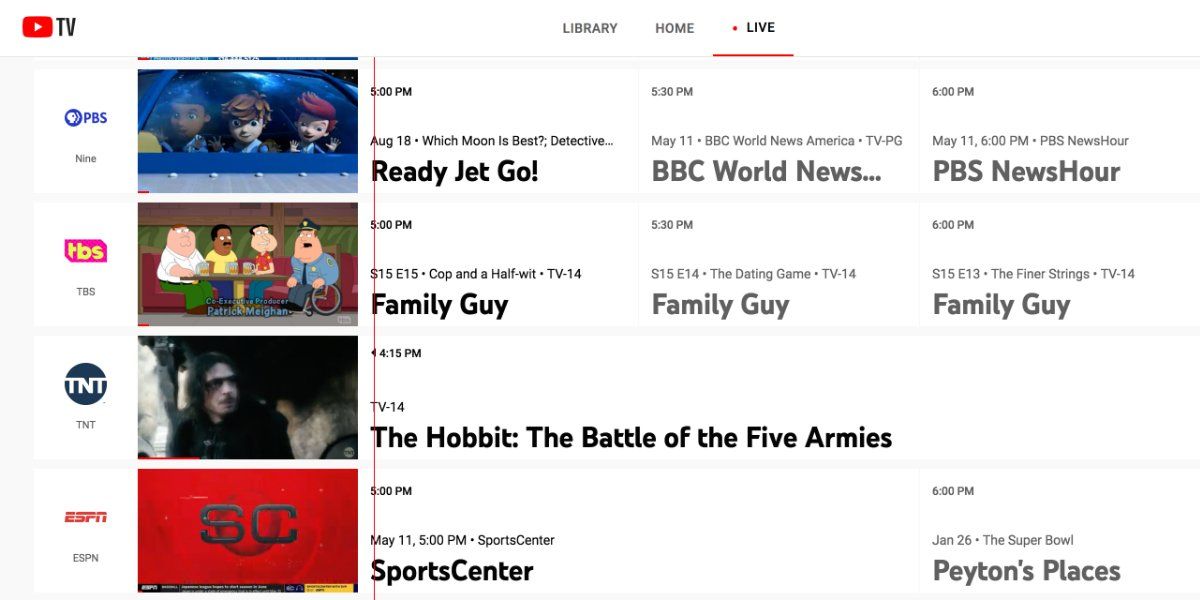**Detailed Caption:**

This image showcases the YouTube TV interface. In the top left-hand corner, there's the iconic YouTube logo—a red play button with a white right-facing arrow—followed by the text "TV." Moving to the right, centrally located at the top, you find the navigation options: "Library" in gray, "Home" in gray, and "Live" in dark gray. The "Live" option also features a red dot next to it and is underlined in red, indicating it is the current selection.

On the left-hand side of the screen, there is a channel list. The first entry shows "PBS" in blue with "9" in gray just below it. Adjacent to this are thumbnails and program details. The first thumbnail depicts a cartoon or claymation image of three little girls sitting in the back of a car.

Next, the channel "TBS" is listed in yellow with a pink flag behind it, with a second "TBS" label in gray underneath. A thumbnail to the right displays an image from "Family Guy," featuring a character sitting at a bar. Just to the right, it shows the air time as "5:00 PM," with episode details "S15, E15, Cop and a Half" rated TV-14 below it, and "Family Guy" written at the bottom. 

Further right, another time block reads "5:30 PM" in black, with "S15, E14, The Dating Game" and TV-14 rating below, followed by "Family Guy." Continuing to the right, the next time slot reads "6:00 PM" with "S15, E13, The Finer Strings" underneath, followed by "Family Guy."

Back on the left side, there's a black circle with "TNT" in white letters, with a smaller "TNT" in gray below it. To the right of this, a thumbnail depicts a very pale-skinned man with shoulder-length dark hair, wearing a black overcoat. The air time "4:15 PM" is listed in black, followed by a TV-14 rating in gray, and the movie title "The Hobbit: The Battle of the Five Armies" in bold black letters.

Continuing to the next channel segment, it shows "ESPN" in red with a smaller "ESPN" in gray below. To the right of this segment is a thumbnail with a red background and a gray circle containing the letters "SC" in gray. Next to it, it reads "5:00 PM" in black, with "May 11, 5:00 PM, SportsCenter" underneath in gray, and "SportsCenter" in bold black letters. Further right, another segment reads "6:00 PM, January 26" with "The Super Bowl" and "Peyton's Places" listed in gray.